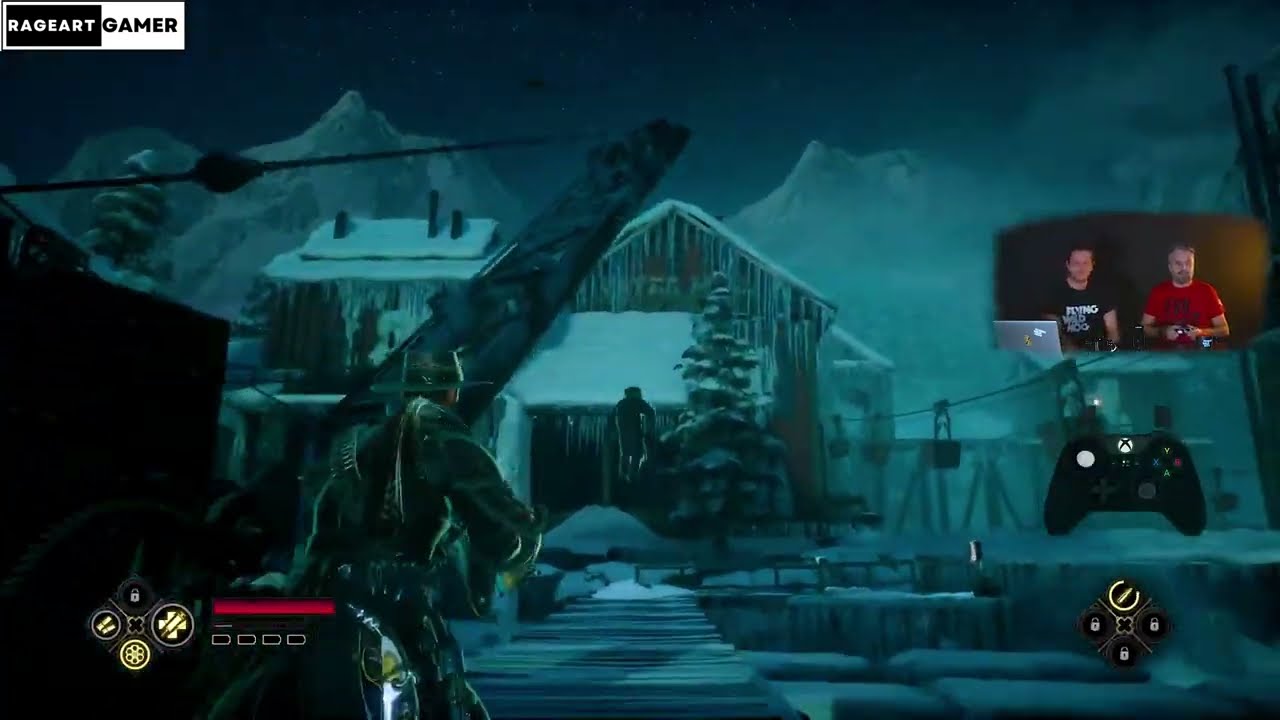In this vivid screenshot, we see an immersive nighttime scene from a video game featuring a snowy setting, possibly viewed through a streaming setup. The background is dominated by towering snow-covered mountains and a cabin draped with icicles. Central to the game scene, a soldier-like character, donned with a cowboy hat and bullet straps, seems to be stealthily navigating a dock. The air of tension is heightened by the lack of light, characteristic of a night-time environment. In the bottom right, a black Xbox controller overlay indicates the platform, accompanied by a set of menu options with lock icons and a life bar, hinting at gameplay elements to unlock. Additionally, a smaller, superimposed webcam feed shows two men at a gaming setup; one, wearing a red shirt, is interacting with the controller, while the other, in a black shirt, observes and manages a nearby computer. In the upper left corner, the text "RAGE ART GAMER" is displayed in black and white, perhaps the streamer's channel name.